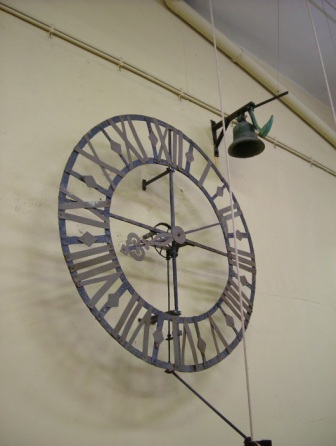A detailed, cleaned-up caption:

"A wireframe clock mounted on a beige wall, situated beneath a projector screen with an attached dark green alarm bell. The clock features Roman numerals from I to XII in a lighter blue color, with wireframe segments connecting the outer circle to the inner circle between each numeral. The inner circle is centered with a plus sign, anchoring the top, bottom, and sides. Clock hands, also in a lighter blue hue, are attached at this central plus sign. The hands, which are in a lighter color, indicate the time as approximately 2:10. The wireframe structure supporting the clock is a contrasting darker blue, providing a subtle yet distinct framework."